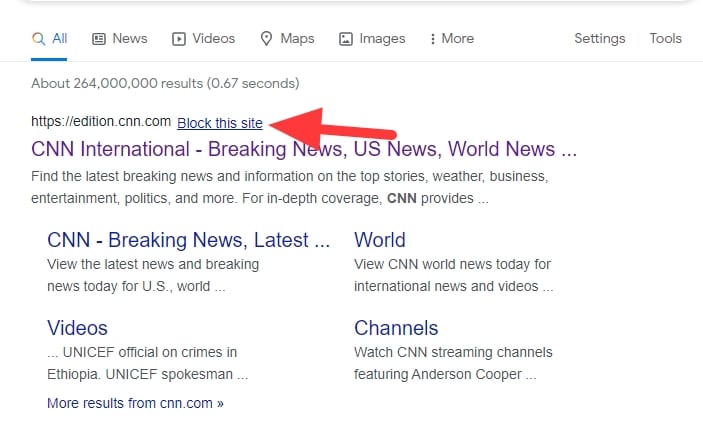The image depicted is a screenshot from a Google search results page. The screenshot starts just below the search bar, with the top portion of the page displaying the standard filter options for search results: All, News, Videos, Maps, Images, and More. The 'All' option is selected, highlighted in blue with an underline, while the other options are grayed out. Alongside these, there are additional options labeled 'Settings' and 'Tools'.

Beneath these, the page indicates that about 264 million results were found in 0.67 seconds. The first search result is from the URL "https://edition.cnn.com," with a prominent blue button labeled "Block this site" and a large red arrow Photoshopped pointing to it. This result is titled "CNN International - Breaking News, US News, and World News," highlighted in purple, indicating it has been visited. The description under the link reads: "Find the latest breaking news and information, top stories, weather, business, entertainment, politics, and more for in-depth coverage CNN provides..."

Below this primary link, there are four smaller, clickable links: "CNN Breaking News," "Latest World," "Videos," and "Channels." At the very bottom, there's a "More results from CNN.com" link, suggesting additional related content from the same website.